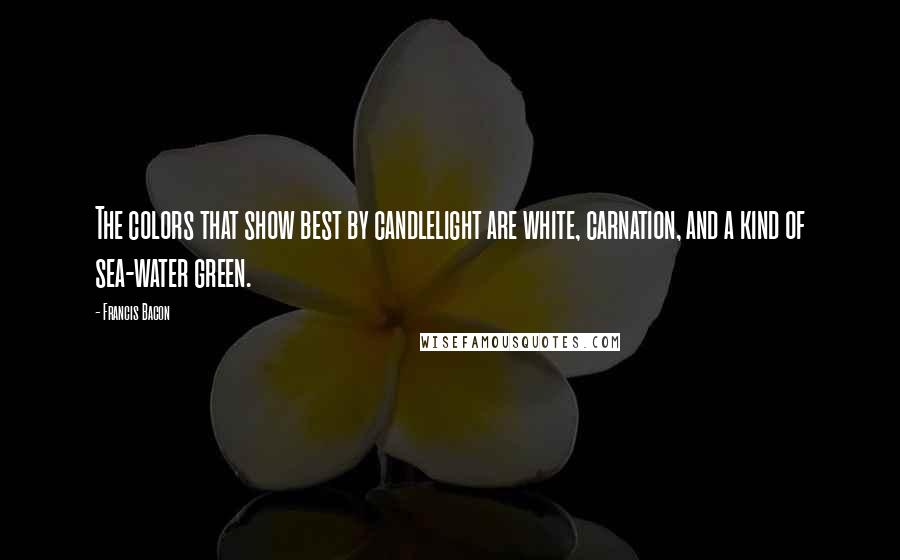The image features a large, somewhat dimmed Hawaiian flower, often used in leis, set against an entirely black background. The flower, which appears white with a yellow and orange center and green leaves near the bottom, is slightly out of focus. Superimposed in white text in the middle of the picture is an inspirational quote by Francis Bacon: "The colors that show best by candlelight are white, carnation, and kind of seawater green." Below the quote lies a faint watermark in black text within a white box, attributing the quote to wisefamousquotes.com.